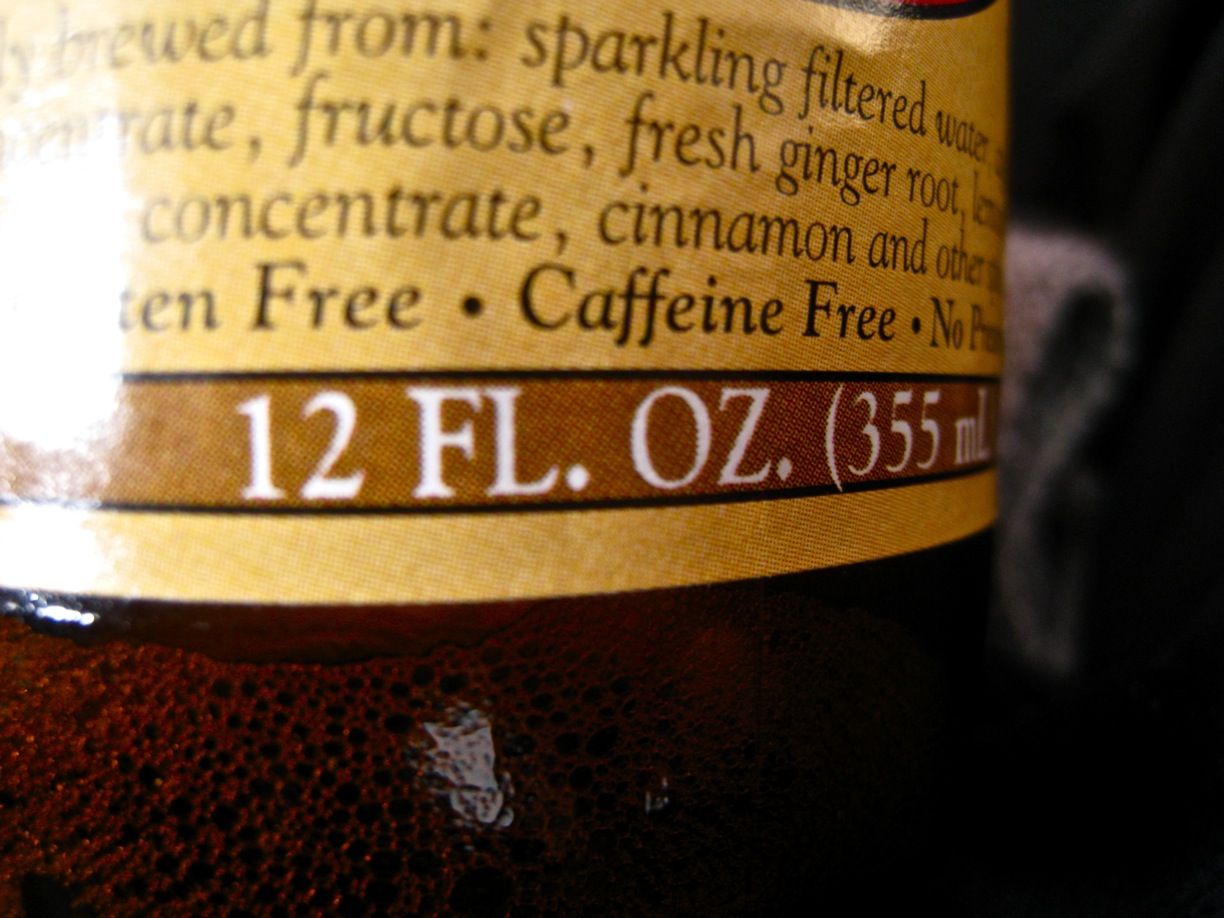This horizontal rectangular color photograph captures an extremely close-up view of a bottle containing a drink. The bottle features a tannish-yellow label that lists various ingredients and specifications. Notable details include the presence of sparkling filtered water, fructose, fresh ginger root, cinnamon, and possibly other concentrates. The bottle is identified as gluten-free, caffeine-free, and containing no preservatives. The liquid inside the transparent glass bottle appears dark brown, resembling coffee with a frothy texture visible near the bottom. Despite a glare on the right side of the label, making some text difficult to read, the visible part of the label confirms the volume as 12 fluid ounces (355 milliliters). The meticulous detail, including ingredients and regulatory marks, suggests it is a carefully crafted beverage meant for consumption.